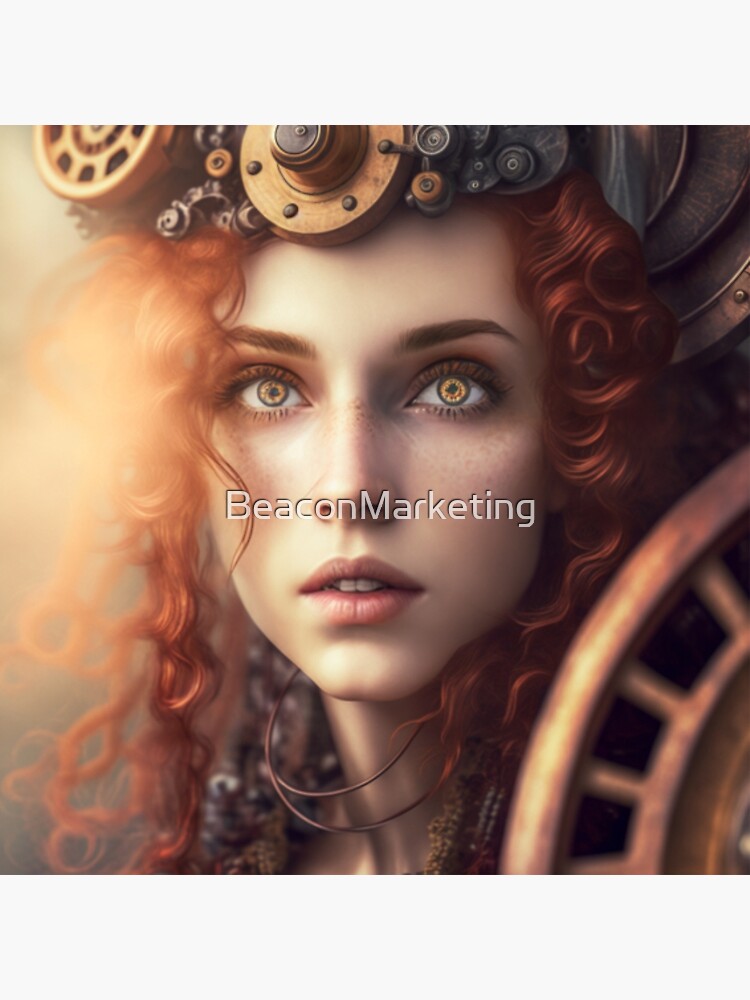The image features a digital or painted portrait of a woman with striking curly red hair and mesmerizing green eyes, although some perceive them as yellow. She is facing straight ahead, and her face, adorned with red lipstick, commands the center of the composition. The portrait bears the text "Beacon Marketing" prominently. Her head is adorned with an intricate headpiece consisting of wheels, cogs, and knobs in hues of gray and bronze, adding a steampunk-like aesthetic. The composition is rich with colors including maroon, red, brown, and subtle highlights of white, with her detailed eyelashes and flowing hair framing her face, focusing the viewer's attention on her enigmatic expression.